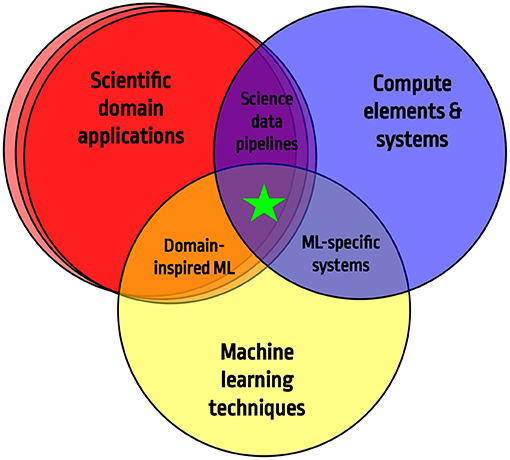The image is an infographic featuring a Venn diagram composed of three overlapping circular disks arranged in a triangular formation, with a red circle at the top left, a blue-violet circle at the top right, and a cream-colored circle at the bottom. Each circle is outlined with a thin black border and contains black text related to machine learning. The red circle, labeled "scientific domain applications," exhibits a pink shadow on its left side. The blue-violet circle is labeled "compute elements and systems," and the cream-colored circle is labeled "machine learning techniques."

In the intersections of these circles, different colors and texts appear to indicate the combination of these domains. The overlap between the red and cream circles forms an orange area labeled "domain-inspired ML." The overlap between the blue-violet and red circles results in a dark purple area labeled "science data pipelines." The convergence of the blue-violet and cream circles produces a lighter purple region labeled "ML-specific systems." At the very center, where all three circles intersect, there is a darker purple area featuring a green star, symbolizing the core intersection of these fields. The entire Venn diagram is set against a pure white background.